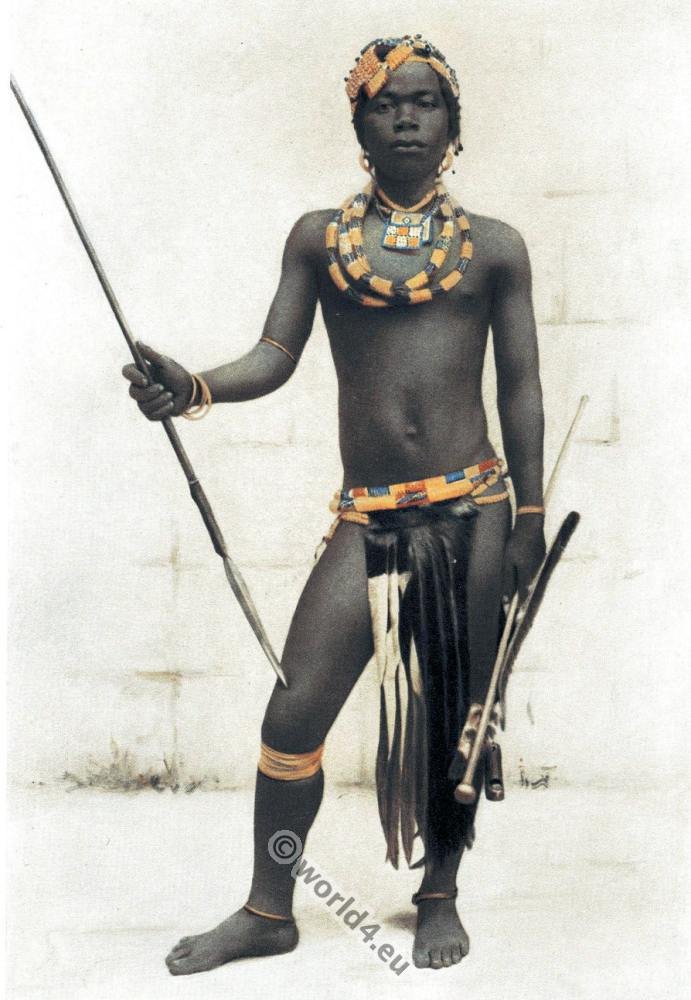This image features an African or African-American male with dark complexion, depicted in a striking, traditional attire. He has a serious, solemn facial expression and is adorned with vibrant jewelry and accessories. Around his neck is a necklace composed of alternating orange and black beads. He wears a decorative orange headband and an intricately beaded belt around his waist, with additional orange cloths draped around his knees and pelvis area. His attire includes ankle bracelets. The man is equipped with a spear in his right hand and holds a large metal rod in his left hand. Feathers or possibly strips of hide hang down from his belt, adding to the elaborate beadwork of his outfit. He stands on a white floor against a brick white wall, presenting a timeless image that exudes cultural richness and intensity.